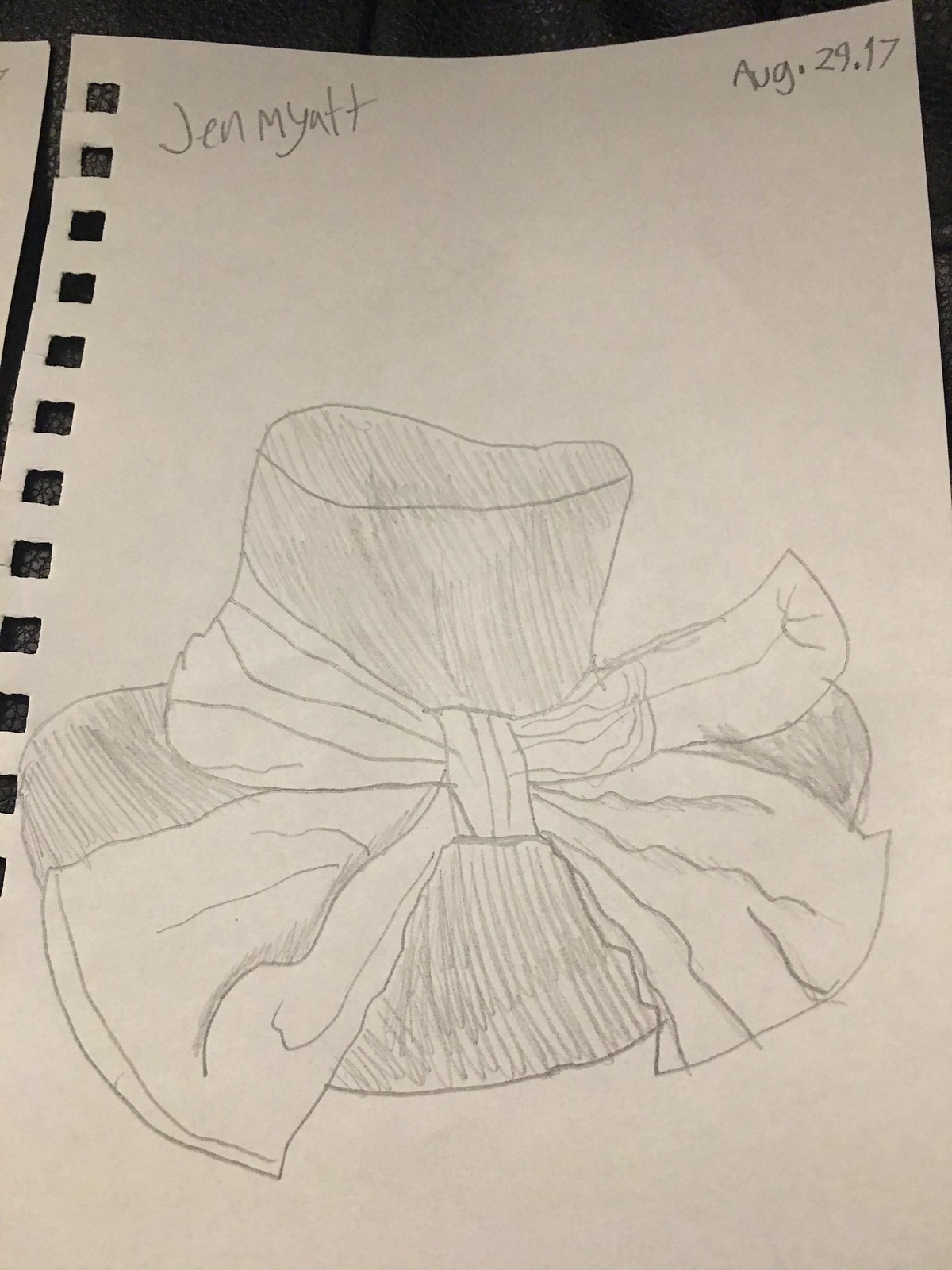The image showcases a detailed, top-down view of a piece of spiral sketch paper that has been torn from its binding, evidenced by the ripped edge and visible square holes along the top. In the top left corner, the name "Jen Myatt" is inscribed in pencil, while the top right corner bears the date "August 29th, '17." Dominating the lower center of the paper is an intricately shaded pencil sketch of a large woman's hat. This hat features an oversized bow tied around its middle, with the extensive ends of the bow extending gracefully over the brim. The bow's left end points to the left, and the right end points to the right. The entire sketch, from the hat to the bow, is meticulously shaded in pencil, adding depth and dimension to the drawing.